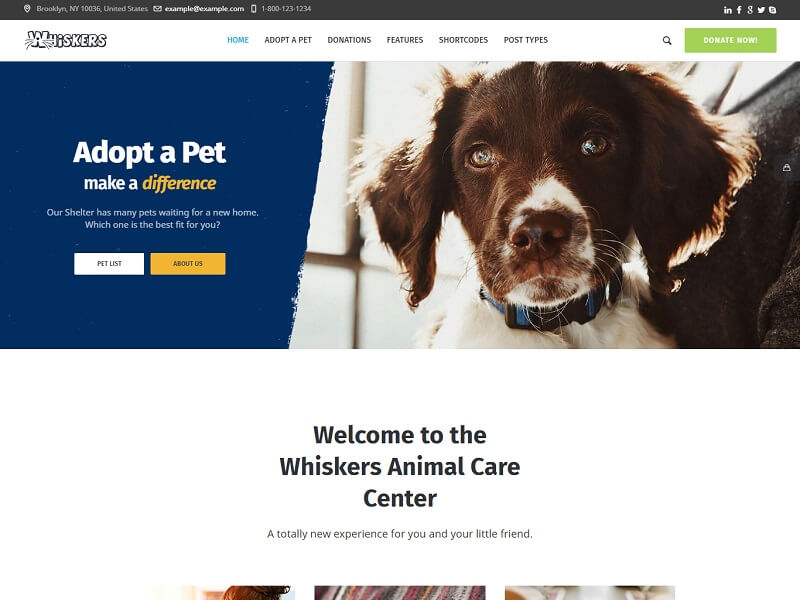The webpage for WHISKERS Animal Care Center features a clean, inviting design tailored to those looking to adopt a pet. In the upper left-hand corner, the name "WHISKERS" is prominently displayed in a playful, bubbly white font with a black outline. A small black bar runs across the top of the page, likely containing crucial contact information such as the location, phone number, and email address of the agency. On the right side of this bar, users can find quick links to the organization’s social media profiles, including Facebook and Twitter.

Dominating the middle to right-hand side of the page is a large, heartwarming image of a dog's face. The dog, wearing a blue collar, has a predominantly brown coat with touches of white on its nose, ears, and chest. This visual is designed to capture the viewer's attention and evoke empathy.

On the left-hand side of the main image, bold text reads, "Adopt a pet, make a difference. Our shelter has many pets waiting for new homes. Which one is best for you?" Below this inviting message, there are two prominent links: "Pet List" and "About Us." Finally, at the bottom of the page, a welcoming message introduces visitors to the Whiskers Animal Care Center, promising "A totally new experience for you and your little friend."